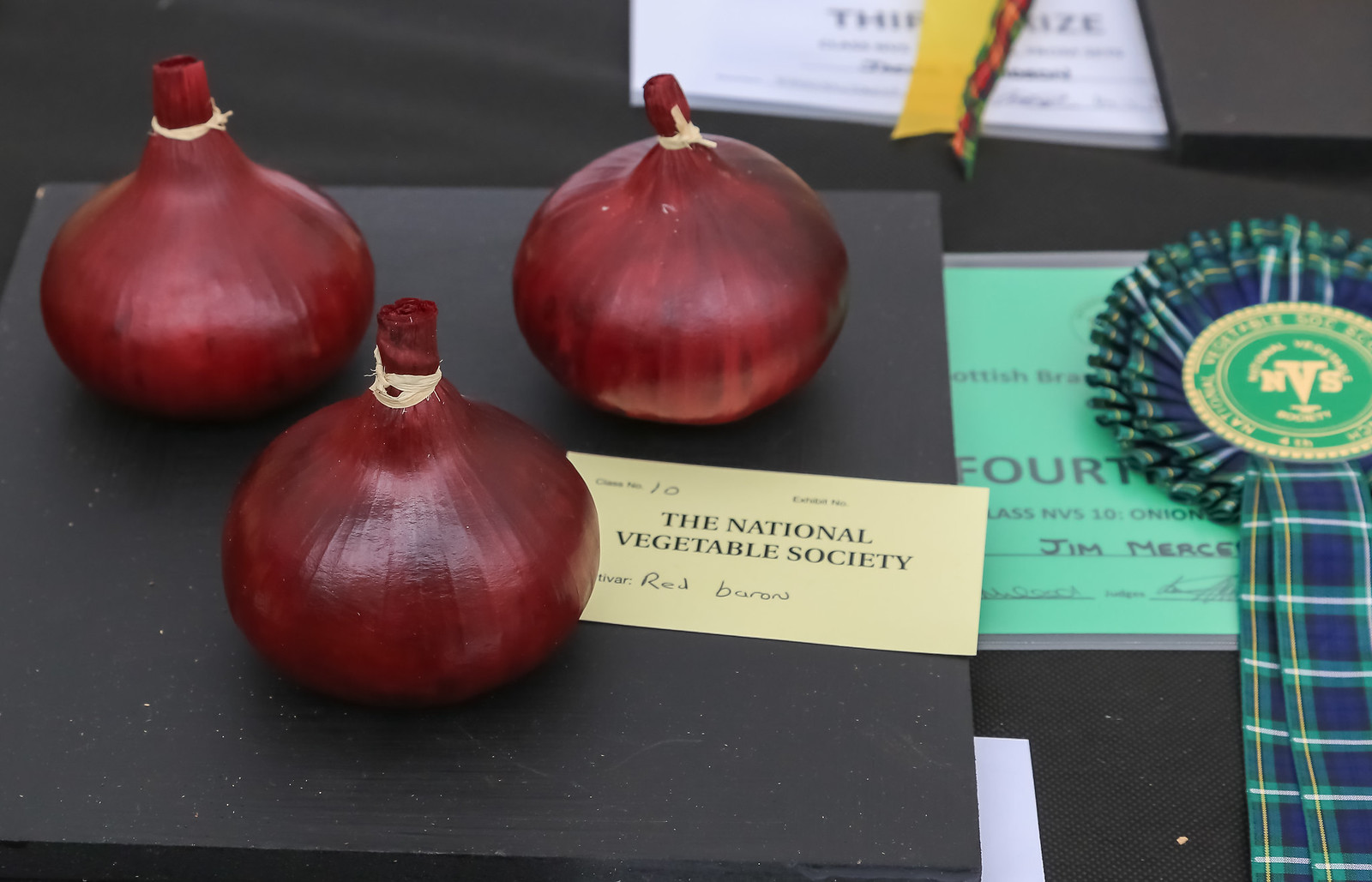The photograph captures a meticulously arranged display, likely from a vegetable judging contest, featuring three deep crimson red onions with perfectly rounded shapes and a waxy appearance. These onions, each with a tied knot at the top, are set on a black tablecloth-covered surface. A prominent yellow card on this table reads "The National Vegetable Society" in black font, with "Red Baron" handwritten below, along with the number "10." To the right of the onions, a blue, green, and yellow award ribbon is visible, adorned with gold fringe and the initials "NVS" prominently displayed in the center. Below the ribbon lies a light green laminated certificate inscribed with "Fourth" and partially obscured text revealing the name "Jim Mercer." The setup includes additional ribbons and signs, indicative of a high-stakes competition, possibly featuring the work of students at a science fair.